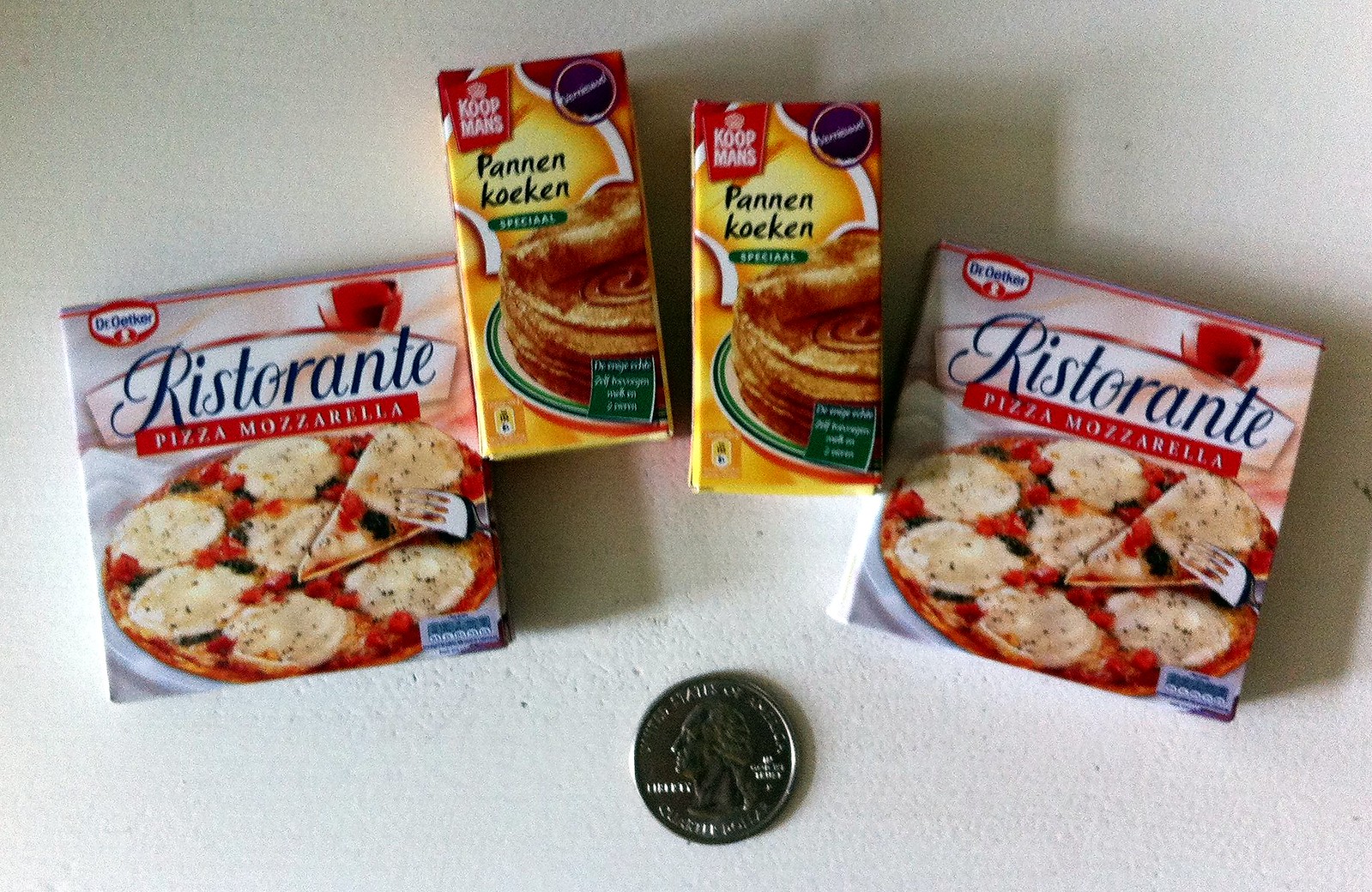The image features an assortment of food products in various packaging. In the foreground, there are two boxes of "Ristorante Pizza Mozzarella," prominently showcasing the brand name "Ristorante" in blue and "Pizza Mozzarella" in red. The packaging displays an appetizing pizza topped with mozzarella cheese, with a fork lifting a piece to highlight its texture and toppings. 

Flanking these boxes on the left and right are identical packs of a different product labeled "Penn in Coke." Although the specific nature of the product isn’t clear, it appears to contain a creamy substance. The Penn in Coke packaging includes a green box situated beneath a yellowish background. 

The top left corner of the frame features a red box labeled "Coopman’s," while the top right corner has a distinctive blue circle. 

Finally, below all the food products, there is a quarter lying on its edge, resting on a white surface that serves as the backdrop for the entire arrangement.